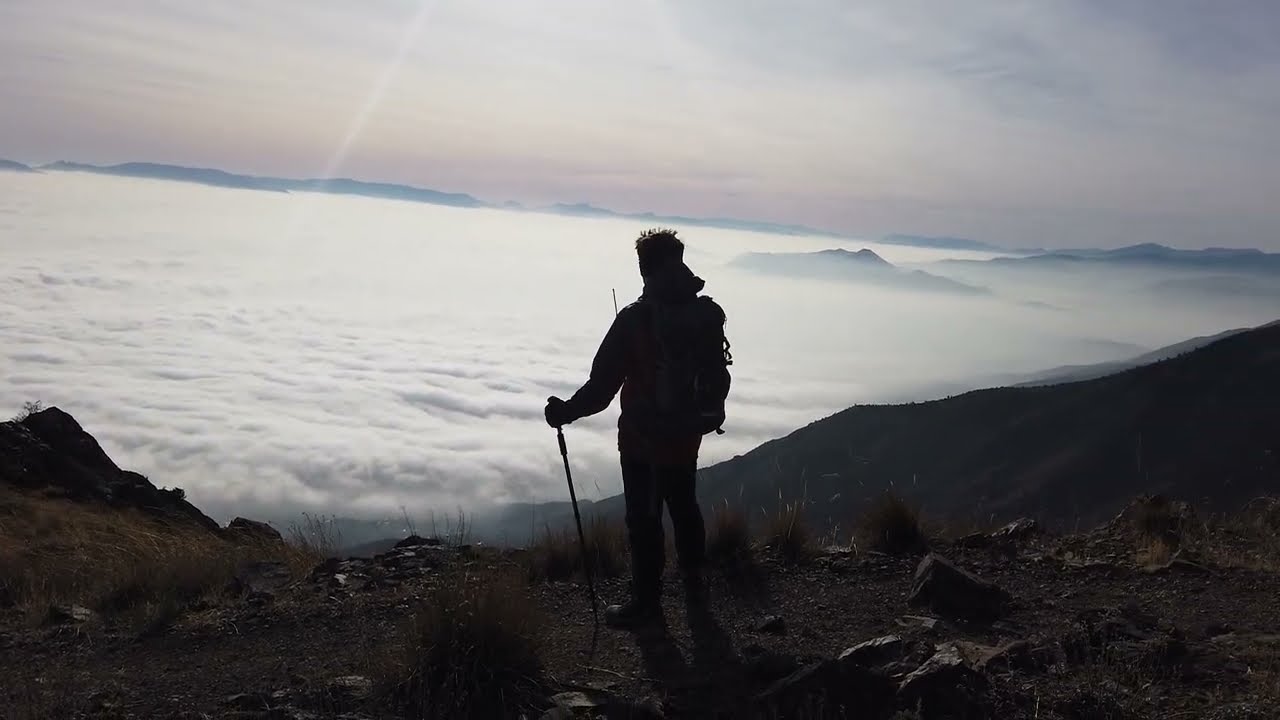The image captures the silhouette of a hiker standing atop a high mountain range, enveloped by the dramatic shadows cast by the nearing sunset or sunrise. This lone adventurer holds a walking stick in his left hand and possibly wears a hooded jacket with a backpack in tow. The foreground is a mixture of mostly dirt, sporadic dried bushes, and rugged rocks, adding to the ruggedness of the scene. The hiker is looking down at the thick blanket of clouds below, with a few mountain peaks piercing through. The sky above is a mesmerizing gradient, transitioning from white at the top to yellow and then a soft pink near the horizon, accentuating the elevated vantage point and the serene yet intense beauty of the moment.